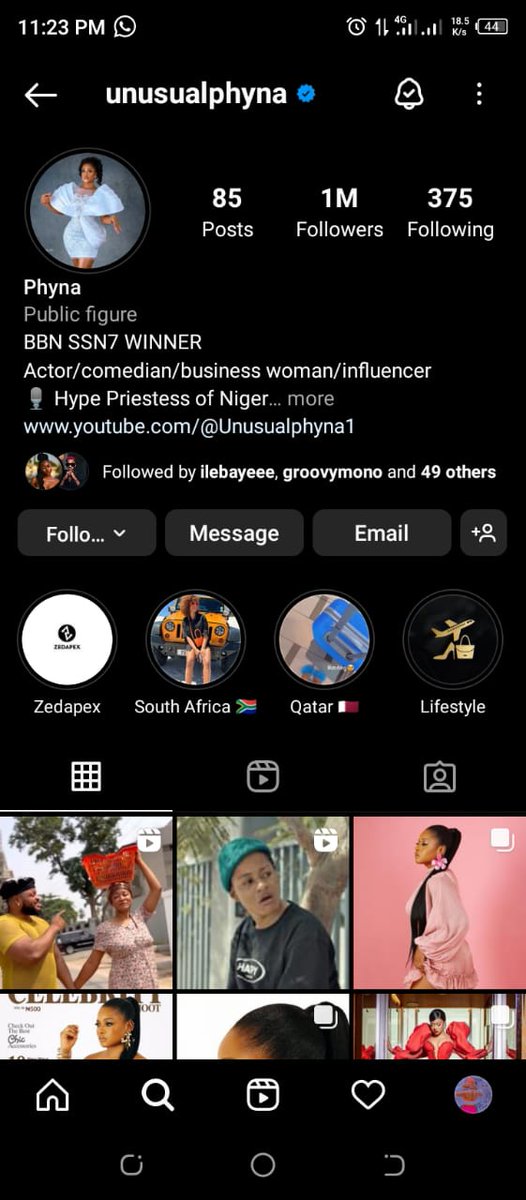This image depicts a screenshot from an Android device taken at 11:23 p.m. The screen is displaying the Instagram profile of a user named "Unusual Phyna," a verified public figure and the winner of BBNaija Season 7. The profile highlights that she is an actor, comedian, businesswoman, and influencer, self-described as the "Hype Priestess of Niger." 

In the header, there is a profile picture of Phyna wearing a short, white poofy dress. The profile boasts 85 posts, 1 million followers, and 375 accounts she is following. The bio section includes a link to her YouTube: www.youtube.com/@UnusualPhyna1. Phyna is followed by notable users such as Ilebaye, Groovy Mono, and 49 others. Below her bio, users have the options to follow, message, email, or add her as a friend. Categories like "Zetapix," "South Africa," "Qatar," and "Lifestyle" are visible as part of her posts.

At the bottom of the screen, the Instagram navigation bar shows icons for a house (home), a magnifying glass (search), a play icon (Reels), a heart (activity), and a user profile icon. The standard Android interface elements, including the back arrow, home circle, and app switcher square, are present.

Additionally, the notification bar at the top reveals a WhatsApp notification and indicates that an alarm is set. There are two cellular service indicators, both showing 4G with three out of four bars of strength, and a data rate of 18.5 KB/s. The battery is at 44%.

This detailed description captures the user's activity on Instagram and the various elements visible on their Android device's screen at that moment.